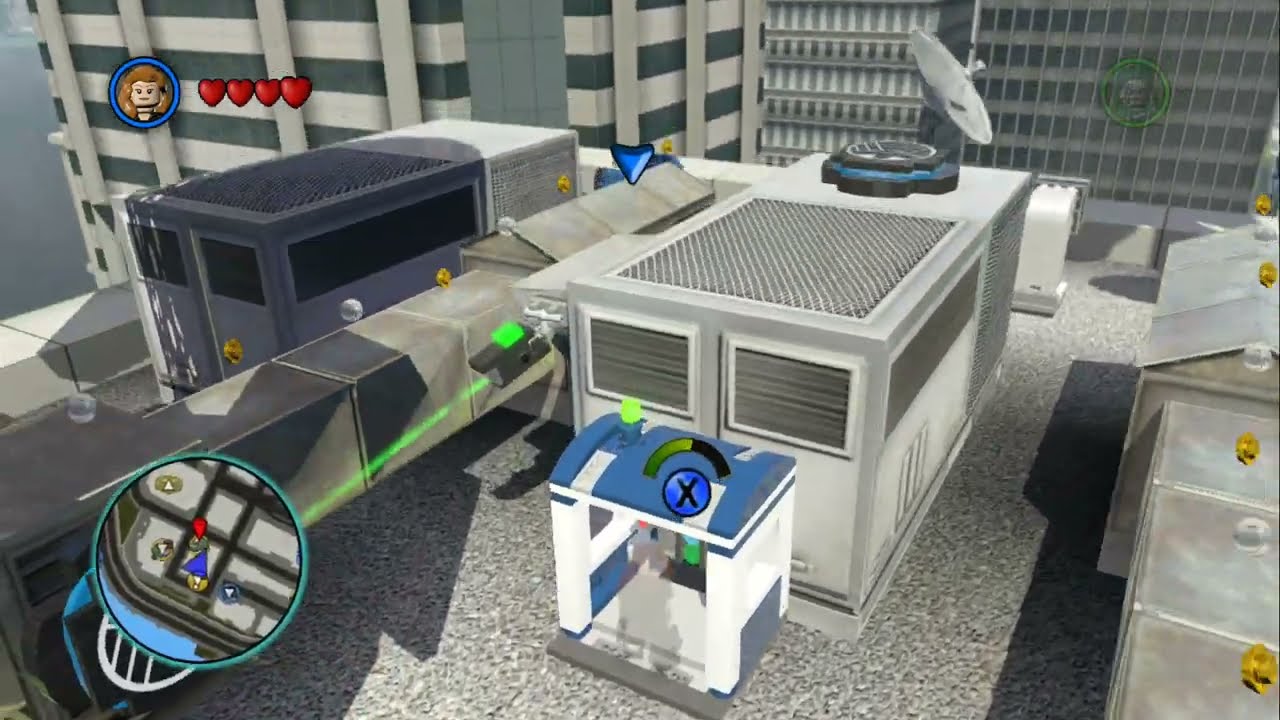This screenshot from a video game captures a vibrant city scene during the daytime. Brick and concrete buildings line the streets, the lower levels housing shops and restaurants adorned with signs above their windows and doors. Characteristic of a bustling urban environment, Lego-like characters populate the sidewalks, going about their day. In front of these buildings, a two-lane street runs left to right, intersecting another street in the foreground. A green vehicle turns right while a blurry yellow car speeds by in the intersection. Lamp posts are visible on either side of the street, casting an orderly charm over the cityscape.

The upper left-hand corner of the image features four black, grayish-white hearts, a common game UI element, alongside a brown-haired character icon within a blue-outlined circle. Contrastingly, the lower left-hand corner shows an inset map with a turquoise border and a directional blue arrow indicating the player’s current location within the game. On the right side of the image, an African American Lego figure with cream-colored hair and a white shirt is partially visible, seemingly walking on the sidewalk.

Noteworthy details include arched windows on the second floor of one large light brown brick building, three distinct shops below, and a mix of street furniture such as green, white, and red streetlights. A staircase to the second floor is also visible in the upper right. The entire street scene, complete with a white building on the left, encapsulates the lively atmosphere of this virtual city.